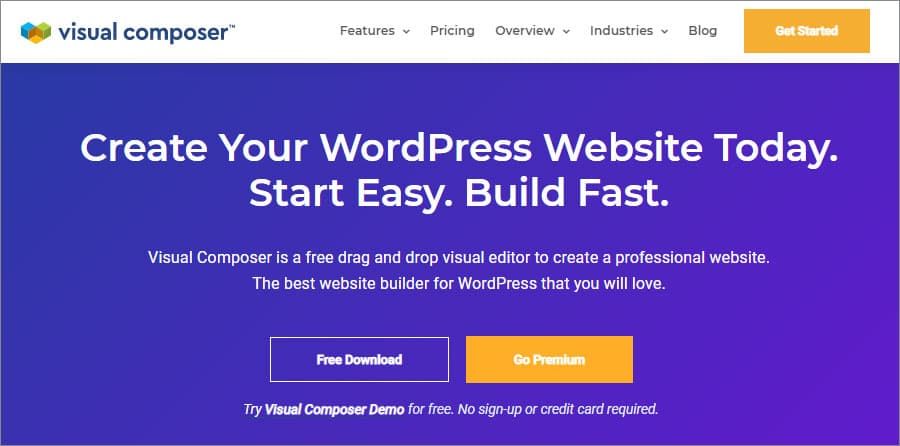The image features a detailed promotional layout for Visual Composer. 

At the very top of the image, there is a narrow white strip adorned with various elements. On the left side, a heart composed of a green box, blue box, and an orange connector stands out. Beneath this heart, the text "Visual Composer" is prominently displayed.

Toward the center of the white strip, there is a navigation menu with the following options: Features (with a pull-down menu), Pricing, Overview (with a pull-down menu), Industries (with a pull-down menu), and Blog. On the far right, an orange "Get Started" button with white font is noticeable.

The background below the white strip transitions into a purple-blue gradient color. Dominating this section in large print are the words, "Create your WordPress website today." Beneath this header, a smaller subtitle reads, "Start Easy, Build Fast." 

Following the subtitle, there is a brief description in much smaller font: "Visual Composer is a free drag-and-drop visual editor to create professional websites. The best website builder for WordPress that you will love."

At the bottom of this section, there are two call-to-action buttons: one matches the background color with a white outline and white font, labeled "Free Download," and the other is an orange button with white font that reads, "Go Premium." Just below these buttons, a line of text invites users with, "Try Visual Composer Demo for free. No sign-up or credit card required."

Throughout the upper white portion of the image, a thin black line borders the left, top, and right edges. However, no line separates the white strip from the purple-blue background.

Overall, the image presents a clean, well-structured, and visually appealing advertisement for Visual Composer's WordPress website building tool.